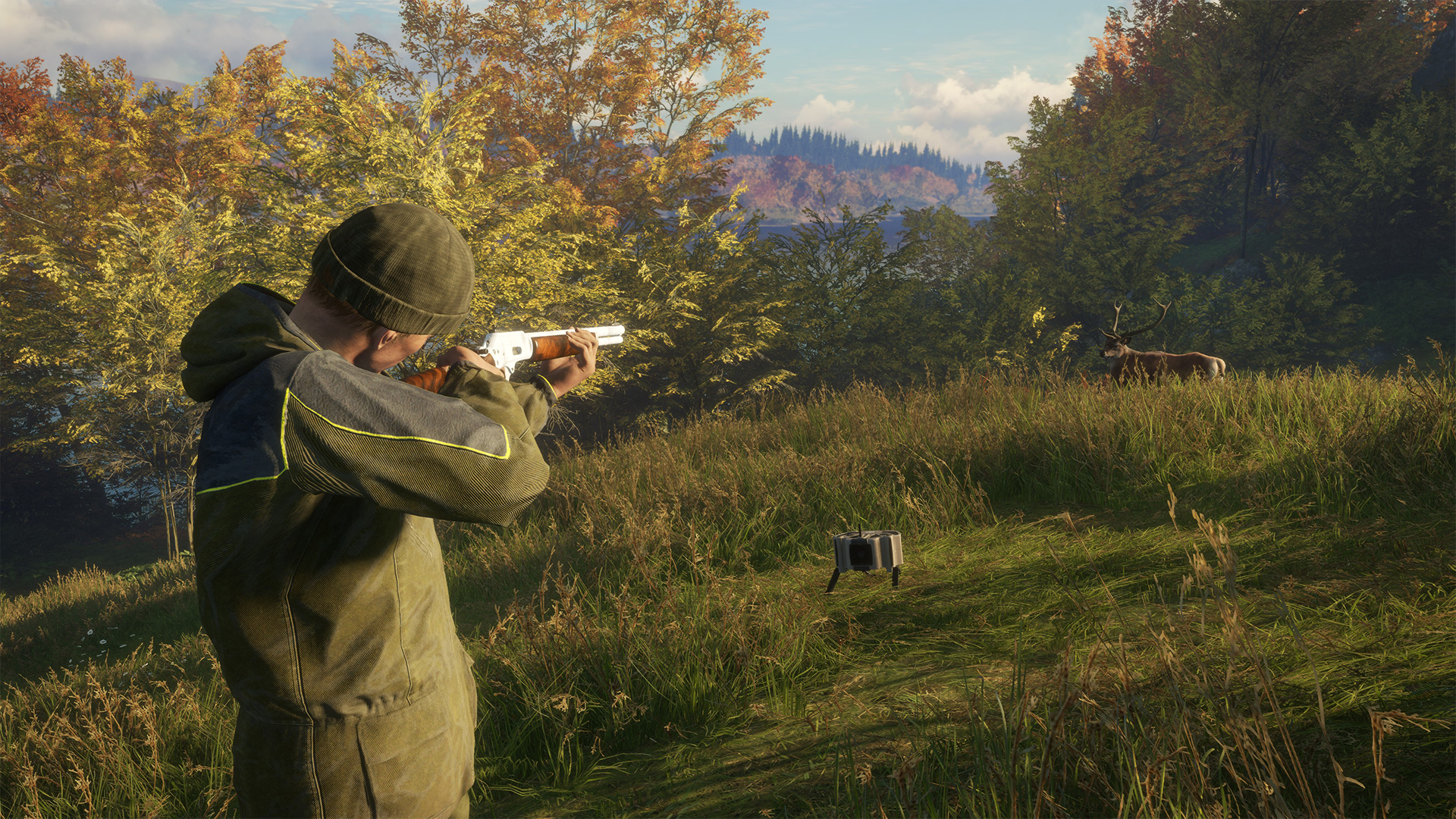In this vivid photograph, a hunter is captured in the midst of taking aim at a very large buck deer. The hunter, dressed in green canvas Carhartt-type attire paired with a camouflage jacket and a green hat or beanie, stands in an open field surrounded by the rich colors of autumn foliage. He is holding a rifle, lining up his shot with focused precision. The scene, set in the late afternoon or early evening as indicated by the sunlight, shows the man on the left side of the image, aiming toward the buck positioned further in the distance on the right. The background features a dense ridge of pine trees, with wispy clouds gracing the sky. The lush countryside comprises both dark and lighter green trees, shedding their leaves which are starting to turn their autumn hues. The setting is picturesque with a small clearing in the grassy area, where a gray metal object, possibly a fire pit, lies in the middle. The buck, which appears to be about 20 to 30 yards away from the hunter, turns its head leftward, seemingly aware of the hunter's presence.